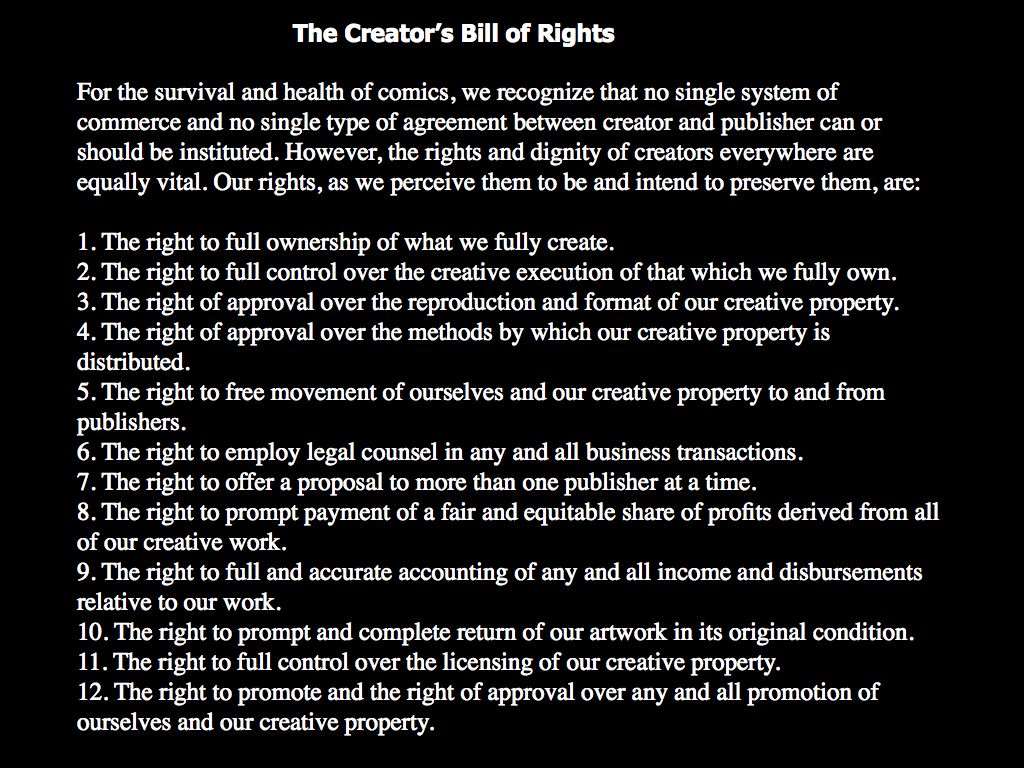This image features plain white text on a solid black background and appears to be sourced from a website or a presentation slide. At the top, in bold white letters, the title reads: "The Creator's Bill of Rights." Below the title, an introductory paragraph states: "For the survival and health of comics, we recognize that no single system of commerce and no single type of agreement between creator and publisher can or should be instituted. However, the rights and dignity of creators everywhere are equally vital. Our rights as we perceive them to be, and intend to preserve them, are:" 

Following this, there is a list of 12 numbered statements, each beginning with "The right to." These rights are detailed as follows:
1. The right to full ownership of what we fully create.
2. The right to full control over the creative execution of that which we fully own.
3. The right of approval over the reproduction and format of our creative property.
4. The right of approval over the methods by which our creative property is distributed.
5. The right to free movement of ourselves and our creative property to and from publishers.
6. The right to employ legal counsel in any and all business transactions.
7. The right to offer a proposal to more than one publisher at a time.
8. The right to prompt payment of a fair and equitable share of profits derived from all of our creative work.
9. The right to full and accurate accounting of any and all income and disbursements relative to our work.
10. The right to prompt and complete return of our artwork in its original condition.
11. The right to full control over the licensing of our creative properties.
12. The right to promote and the right of approval over any and all promotion of ourselves and our creative property.

This detailed declaration emphasizes the essential rights necessary for the well-being and independence of comic creators in an industry with diverse commercial practices and agreements.